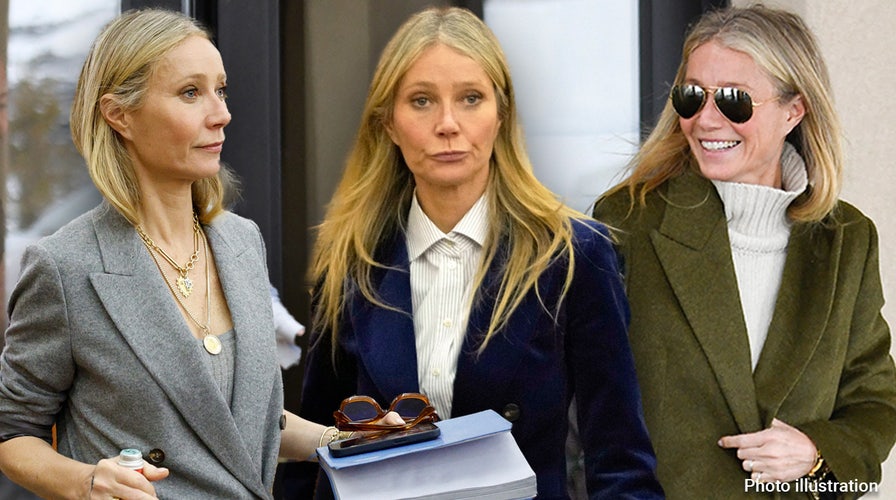The composite image features three separate photos of Gwyneth Paltrow, each showcasing her in distinct outfits and poses. In the left image, Gwyneth is captured from a side angle, wearing a gray top beneath a wool blazer paired with gold necklaces. Her long blonde hair is tucked behind her ear and into her jacket. In her left hand, she holds a phone, books, and sunglasses, while in her right hand, she carries a bottle. The central image portrays her directly facing the camera with a less-than-happy expression, dressed in a white striped dress shirt under a dark blue or velour blazer. Lastly, the right-side image shows Gwyneth smiling brightly while wearing reflective aviator sunglasses. She is dressed in a white cowl neck or mock turtleneck sweater beneath a loose-fitting, mossy green blazer, and she is turning her head to the right. Overall, the images collectively highlight Gwyneth's varied wardrobe choices and her transition from serious to cheerful demeanor.